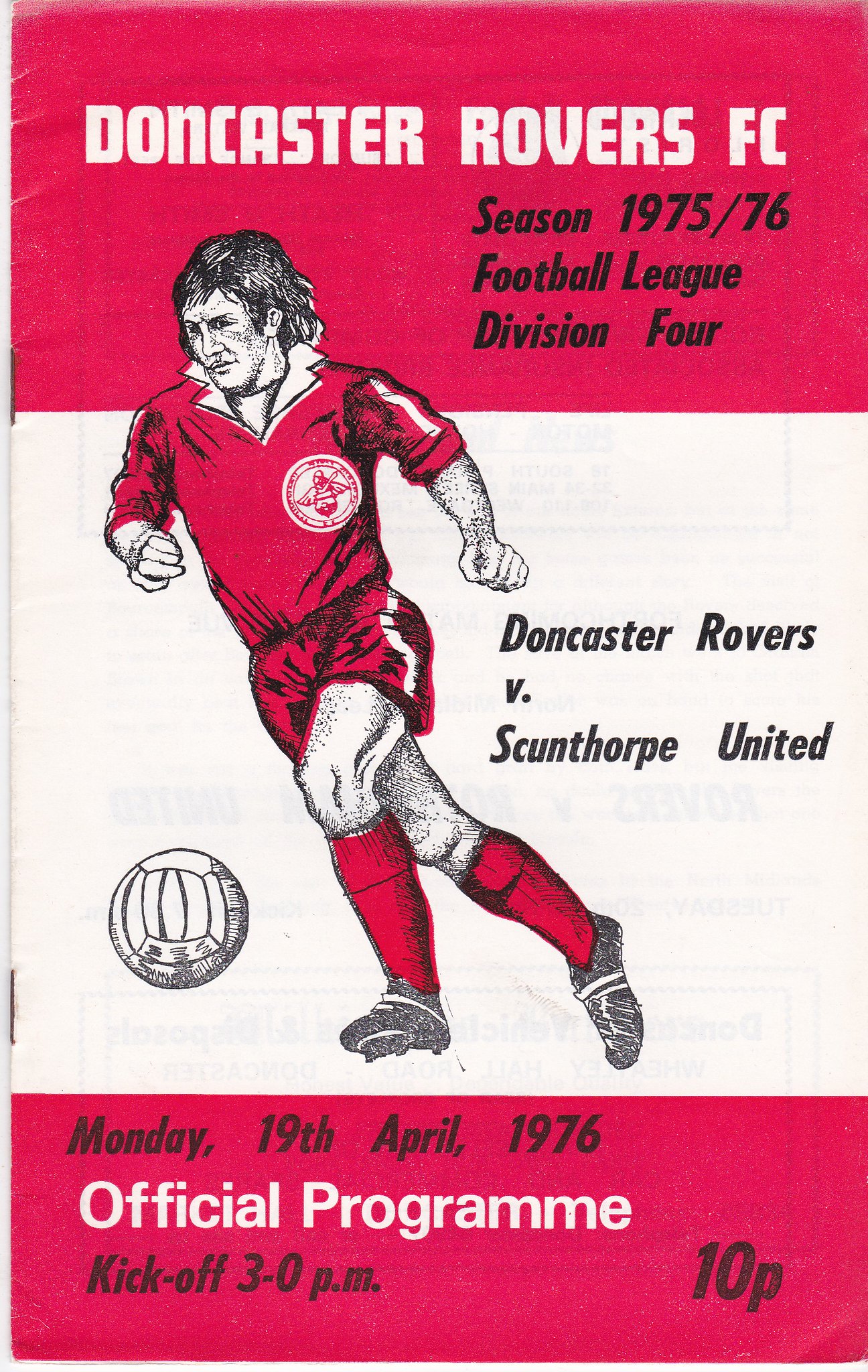This image appears to be the cover of a vintage soccer program for a match between Doncaster Rovers FC and Scunthorpe United in the 1975-1976 Football League Division 4 season. The program cover features a stylized drawing of a man with slightly long hair, dressed in a red and white uniform, captured in mid-action as he runs and kicks a soccer ball. The ball is designed in a traditional black and white pattern, though it might resemble a volleyball to some. The background of the cover is divided into three sections: red at the top and bottom, with white in the middle. At the top, in prominent white lettering, it reads "Doncaster Rovers FC," with the season and league information—"Season 1975-1976 Football League Division 4"—displayed in black below that. The central section indicates that this is an official program for the match, scheduled for Monday, 19th April 1976, with a kickoff time of 3 p.m. At the very bottom, the price of the program is listed as "10 pence (10p)" in the bottom right corner. The program is bound by two visible staples along the left margin, indicating that it is a smaller, stapled booklet.